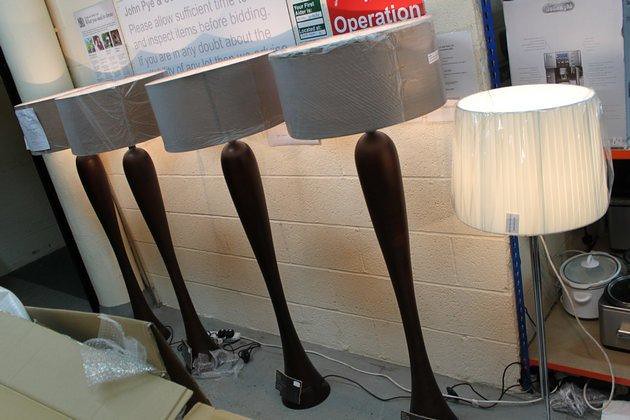This photograph captures an eclectic display of lamps in what appears to be a store, potentially a secondhand or consignment shop. Dominating the scene are four modern, contemporary floor lamps with long, tapering wooden stems that widen slightly at the top before flaring out at the base. These lamps are each adorned with light grayish beige lampshades, and all are turned on, casting a warm light against a predominantly white backdrop with a faint brick texture. Accompanying them is a single mismatched lamp featuring a silver metal stand and a pleated white lampshade, also illuminated. Positioned slightly shorter than the wooden lamps, its top aligns just below the lampshades of the others. Scattered around the base of these lamps are various store items, including a red sign, boxes with bubble wrap, and what appear to be electrical slow cookers, adding to the eclectic and functional ambiance of the store environment. The flooring beneath is a simple gray concrete, grounding the diverse elements within the frame.